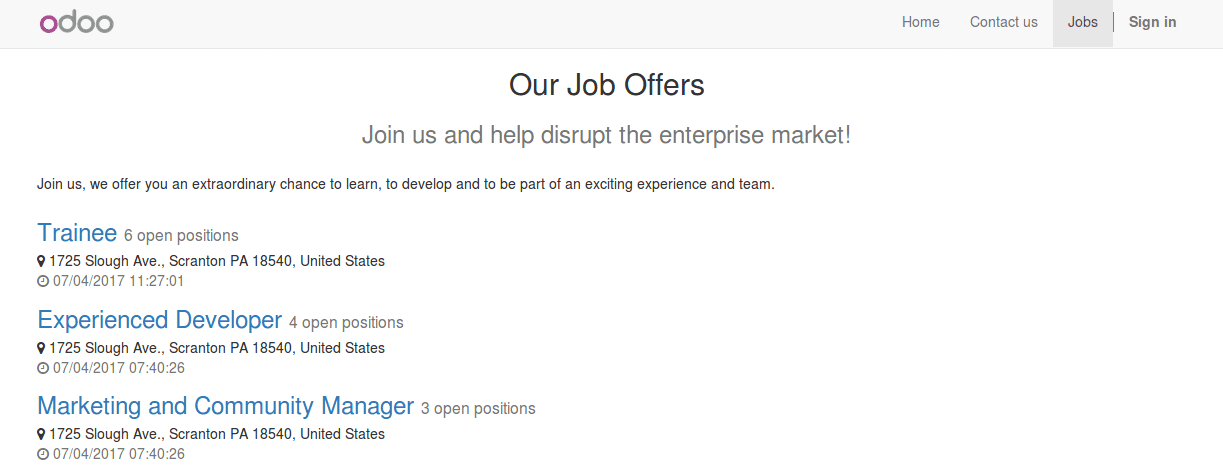The image from the Odoo website prominently features the brand name "odoo" in lowercase letters, with the 'O' displayed in a purplish-pink hue and the remaining letters 'd', 'o', and 'o' in gray. The top area of the page is highlighted by a broad gray rectangle. On the right side of this section, navigation options are listed: "Home," "Contact Us," "Jobs," and a "Sign In" button.

Centered on the page, there is a bold heading that reads "Our Job Offers" followed by an enthusiastic invitation: "Join us and help disrupt the enterprise market!" This is further emphasized with an exclamation point. Below, a subheading encourages potential applicants: "Join us; we offer you an extraordinary chance to learn, develop, and be part of an exciting experience and team."

In the job listings section, details about available positions are presented in blueprint style. It begins with "Trainee," indicating six open positions, and provides a specific location: Scranton, Pennsylvania, United States, along with the date July 4, 2017, and the corresponding time. Following this, two additional job roles are listed — "Experienced Developer" and "Marketing and Community Manager" — both highlighted similarly in blueprint.